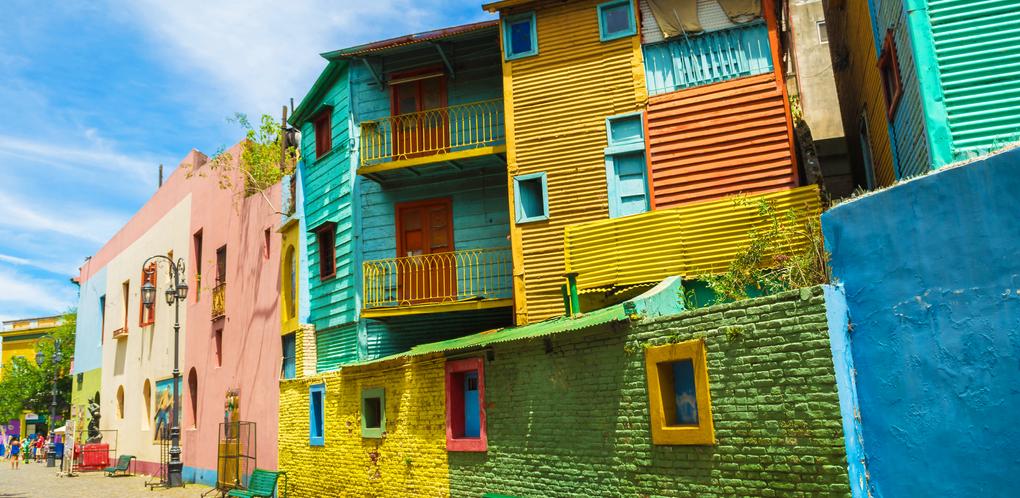This vibrant horizontal photograph captures a vividly colorful block of buildings, reminiscent of tropical or South American architecture. Each building showcases a unique palette and texture, with striking combinations of different colors and materials. A royal blue house stands out with its bright hue, while a green brick wall adorned with a golden-yellow and red window adds a striking contrast. Another building features a red-painted yellow brick facade with royal blue and green windows. Above these, a yellow house with blue windows and a bluish-green house with red doors and windows create a lively scene. A charming pink house boasts a gold balcony, and there's a distinctive white wall with balconies, transitioning from light blue at the top to green at the bottom. The streetscape is completed with a black streetlamp featuring three lanterns and an elevated deck with some plants. The overall composition is rich with yellows, greens, pinks, and blues in various shades and textures, creating a beautiful and picturesque village that looks perfect for photographs or as a vibrant place to live.